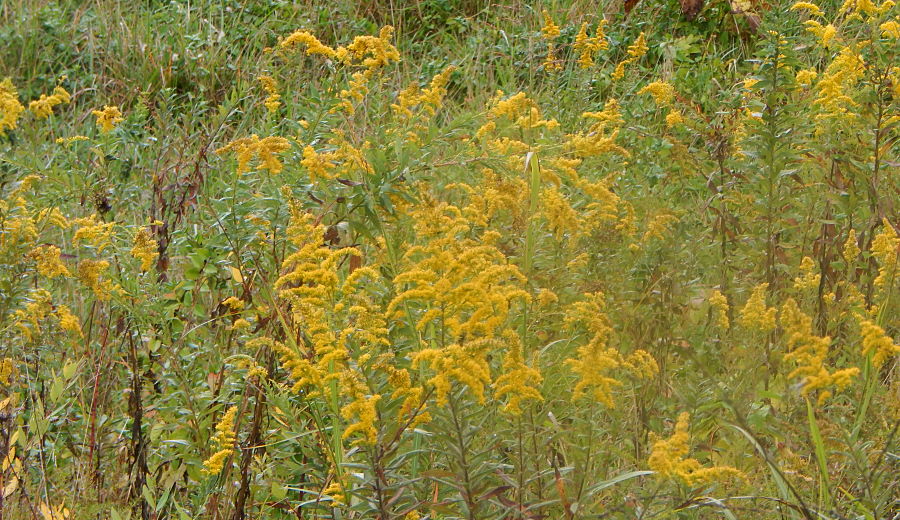The image captures an overgrown field teeming with weeds, tall grasses, and yellow wildflowers. The field is dominated by fluffy, finger-like yellow blossoms that resemble canola, though they appear more like weeds with bunched stems supporting leaves. A mix of green shades highlights the thriving vegetation, with brown, decaying plants interspersed, indicating a late summer or early fall setting. The foreground is dense with greenery and brown stems, while the background merges into a blur of green trees. The overall scene illustrates nature's wild, untamed beauty, emphasizing textures from tall, thick-stemmed weeds to dying grass, presenting a chaotic, yet harmonious landscape.